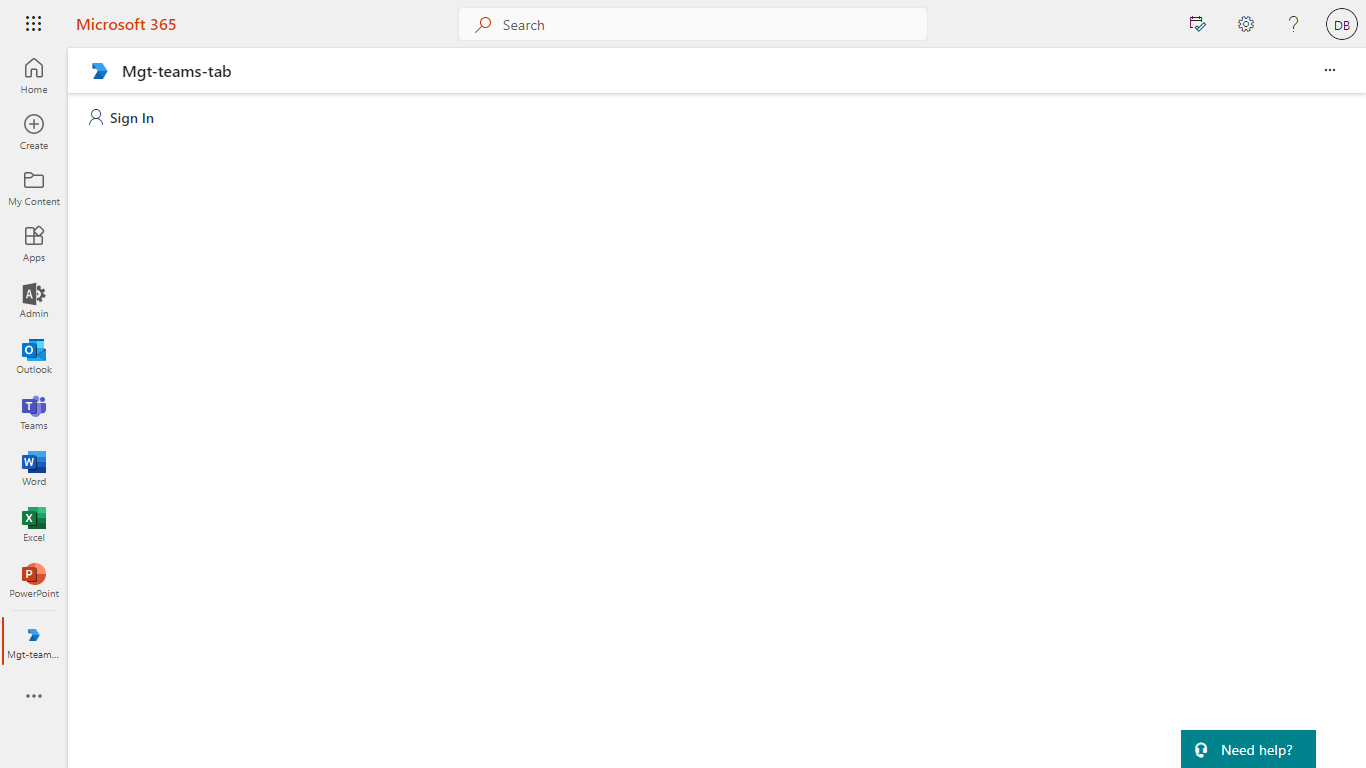The image displays a Microsoft 365 interface window. In the top left corner, there are nine dots arranged in a grid pattern, signifying the app launcher or menu. To the right of these dots, the text "Microsoft 365" is prominently displayed in red. Adjacent to this, there is a white square icon, followed by a magnifying glass icon representing the search function. Further along, there is a gear icon, which is usually indicative of settings. 

Moving to the right, the interface shows the letters "D, D," though their specific function isn't clear from the description. On the far left side of the interface, there is a navigation panel with options labeled: "Home," "Create," "My [something]" (unclear), "Apps," "Admin," "Outlook," "Teams," "Word," "Excel," "PowerPoint," and another unclear option.

Within this interface, a tab header labeled "Management Teams" appears, along with a sign-in option. Additionally, there is an ellipsis (...), often used to indicate more options or settings. The background of the window is predominantly white, providing a clean and minimalist look.

In the central area, there is a large blue rectangle with the text "Need help?" indicating a help or support section. The left side primarily showcases various Microsoft 365 products, emphasizing the suite's diverse application offerings.

Overall, the interface is characterized by clear, predominantly white backgrounds and organized text/font, ensuring ease of navigation and use.